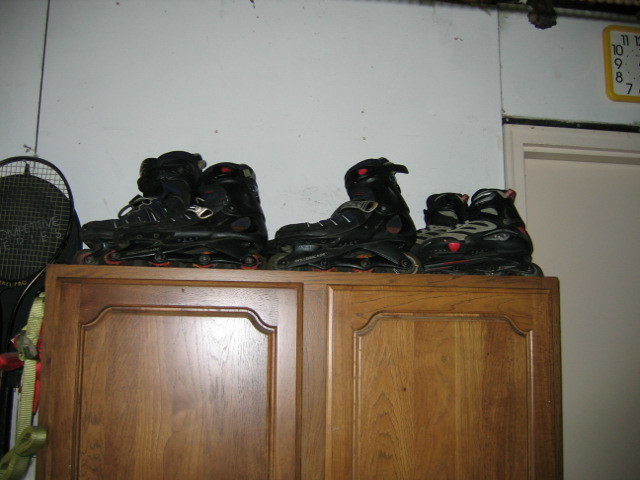This indoor color photograph captures a cabinet, possibly situated in a garage or bedroom, against a white wall. The wooden cabinet, which has detailed curves and grooves, houses a collection of inline skates atop it. There are four pairs of skates; three are predominantly black with some having gray or red details, and one in the middle is a single black skate. To the left of the cabinet is a tennis racket hanging on the wall, alongside a green ribbon. In the right-hand corner, there is a door with a cream-colored frame, and above it, a white clock with yellow trim displaying the numbers 7 through 11, though the hands are not visible. The scene hints at an area designated for sports equipment.